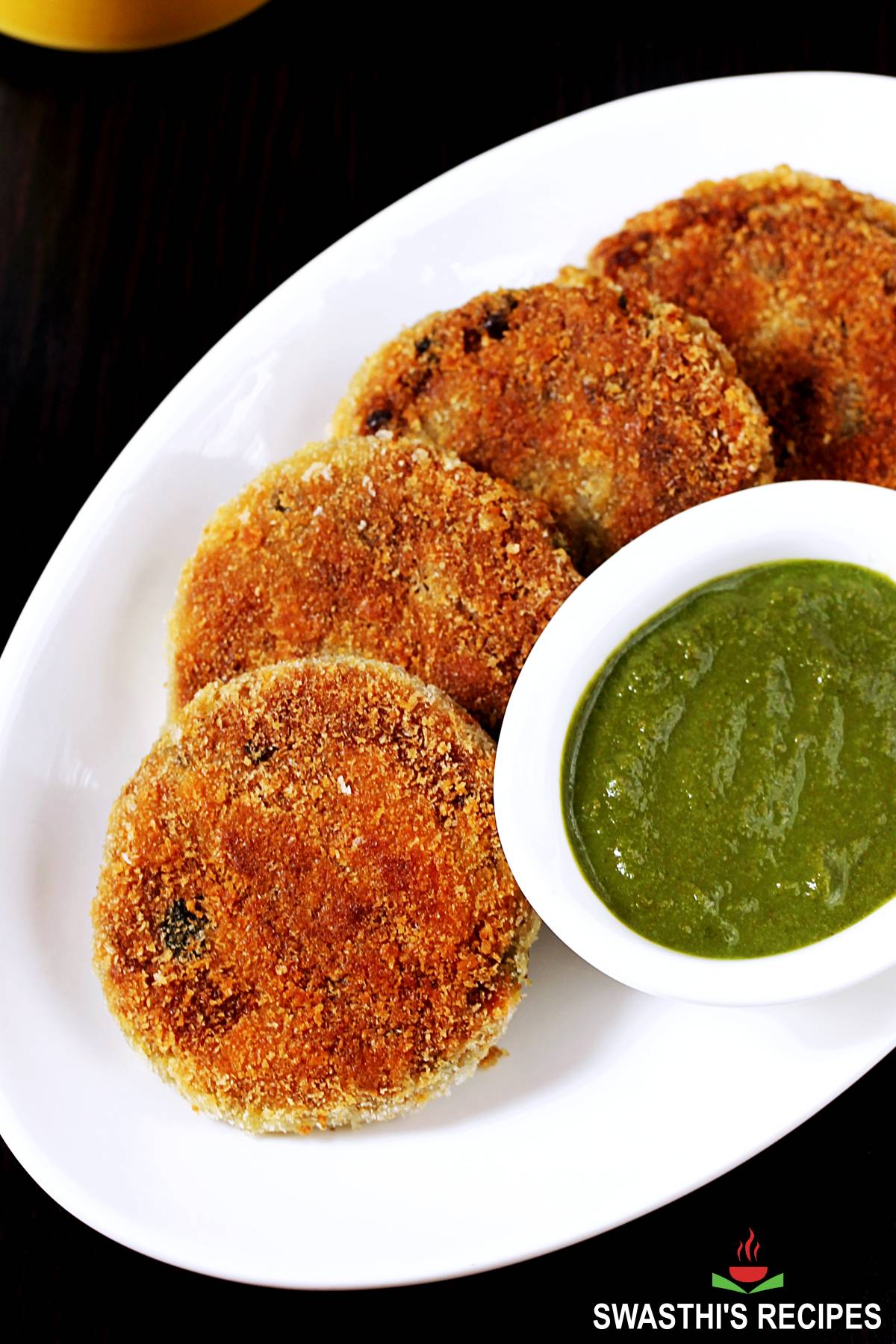This photograph, set against a black background, features a meticulously presented food arrangement. Central to the image is a sleek white oval plate holding four round, golden-browned, breadcrumb-coated fried pieces, which might be eggplant or crab cakes. They are uniformly sized and crisply fried to perfection. To the right of these delectable pieces is a small white bowl containing a rich, creamy green sauce. In the bottom right corner, there's a red bowl emitting steam lines, with "Swathi's Recipes" elegantly printed below in white text, suggesting a hot and tantalizing dish. The careful composition and vibrant colors indicate this is a professional food shot, possibly for a website or a culinary advertisement. Practical details enhance the visual appeal, including a yellow mug peeking from the upper left corner, all contributing to a well-rounded and appetizing display.